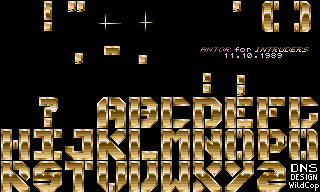Image Description: This is a small, visually striking advertisement set against a black background. Positioned prominently in the center is the English alphabet, each letter meticulously designed in varying hues of dark and light gold. The meticulous gradient and sheen create an eye-catching contrast with the black backdrop. Above these golden letters, abstract shapes can be seen, which do not form any recognizable characters but add an artistic element to the image.

At the lower center of the image, the barely legible phrase "Avaton for intras" hints at either a brand or tagline, adding an enigmatic touch. A date stamp of "11-10-1989" is also present, suggesting a significant event or release date related to the advertisement. 

In the bottom right corner, the text "DNS, Designed Wild Cop" is inscribed, possibly indicating the designer or the studio responsible for the artwork. The black background also subtly features two gold crosses, adding another layer of complexity and visual interest to the overall composition. The image is not only aesthetically appealing but also rich with various elements that invite closer scrutiny.